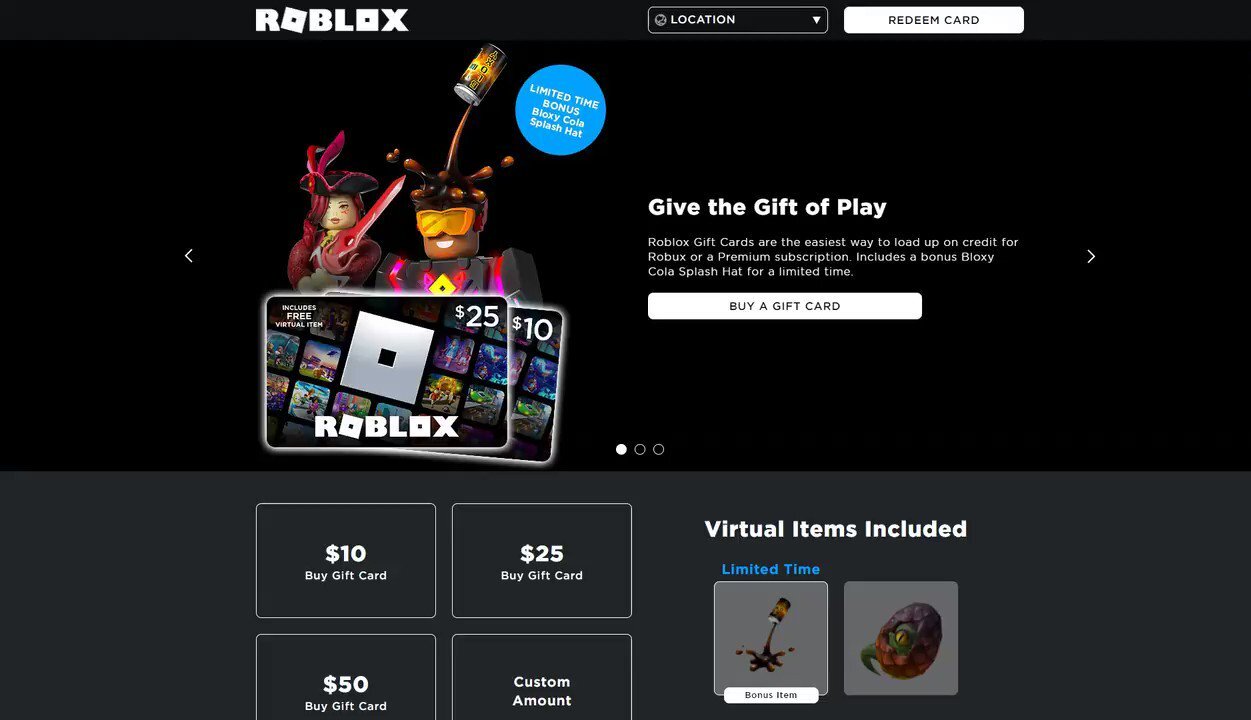The image features a sleek, black background with various elements promoting Roblox gift cards. In the top left corner, "ROBLOX" is prominently displayed in white letters. Below this, there is a black button labeled "location" accompanied by a down arrow, next to a white button that reads "redeem card." On the left side, a small arrow points to an image of two robotic figures resembling a pirate and a joker.

Above these robot figures, a blue circular label announces a "limited time bonus" featuring Bloxy Cola Splash Hat. To the right of the figures, two Roblox gift cards are displayed, one for $25 and another for $10, along with the promotional text "Give the Gift of Play." The accompanying message explains that Roblox gift cards are the easiest way to load up on credit for Roblox or a premium subscription, and includes the mention of the limited-time bonus Bloxy Cola Splash Hat.

Below this promotional content, there is a prominent white button labeled "Buy a Gift Card," accompanied by a right-facing arrow. Towards the bottom of the image, three dots are visible with the first dot filled in white, indicating a selection.

In the lower right section of the image, a large dark gray box is divided into four smaller sections, each containing different gift card amounts: $10, $25, $50, and a customizable amount. The phrase "virtual items included" is mentioned, with a blue "limited time" label. It also shows two squares with additional bonus items; the first depicts a beverage being poured, while the second features an egg-shaped character colored in brown and orange.